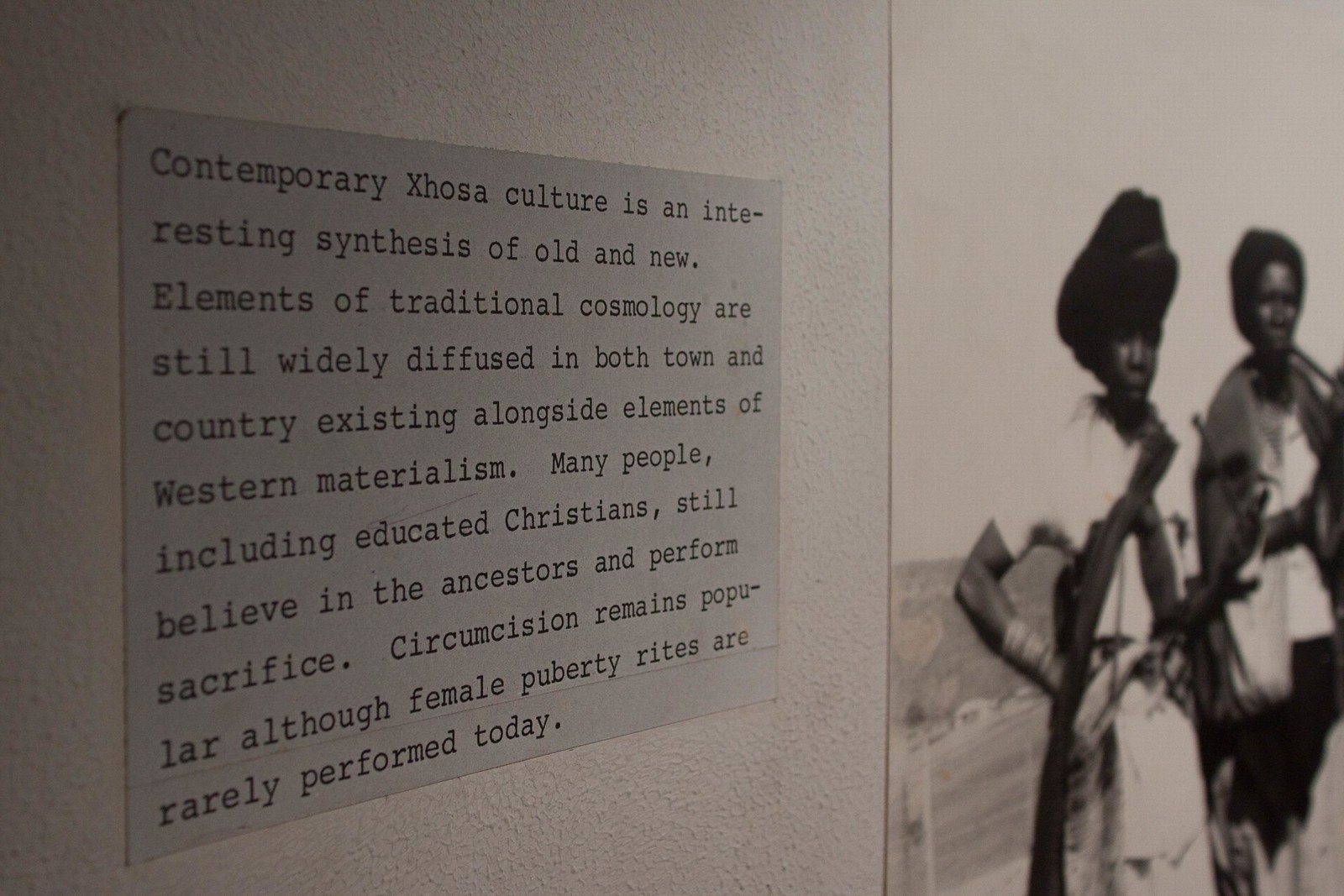The image depicts a museum exhibit featuring a juxtaposition of text and photograph mounted on a wall. On the left, a piece of paper or plaque in a serif font, resembling Times New Roman, provides an in-depth explanation of contemporary Xhosa culture. The text describes how this culture represents a synthesis of old and new elements, blending traditional cosmology with aspects of Western materialism. It details that many people, including educated Christians, continue to honor ancestral beliefs and perform sacrifices, although female puberty rites are now rare. Circumcision, however, remains common.

To the right of the text, a black-and-white photograph is displayed, capturing two African-American women, who appear to be teenagers dressed in traditional cultural garb. Despite the photograph's subtle blur, which keeps it from being the focal point, it adds a visual context to the informative text, highlighting the blend of tradition and modernity within contemporary Xhosa culture.